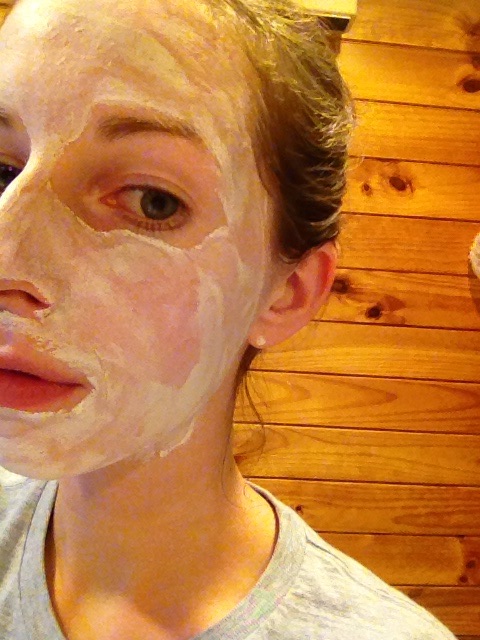In this image, a young Caucasian woman, likely under 30 years old, is seen partially framed against a medium-colored wooden wall, suggestive of a spa, sauna, or wood-paneled bathroom. Her light brown hair is pulled back, possibly in a bun or ponytail, revealing small, round earrings. The photograph only shows her left profile, with half of her face extending out of the frame. She has a white facial mask applied, carefully avoiding the areas around her eyes, lips, and nostrils. Her neck is bare apart from the facial mask extending to the start of it, and she is wearing a light gray t-shirt. There is no text in the image.